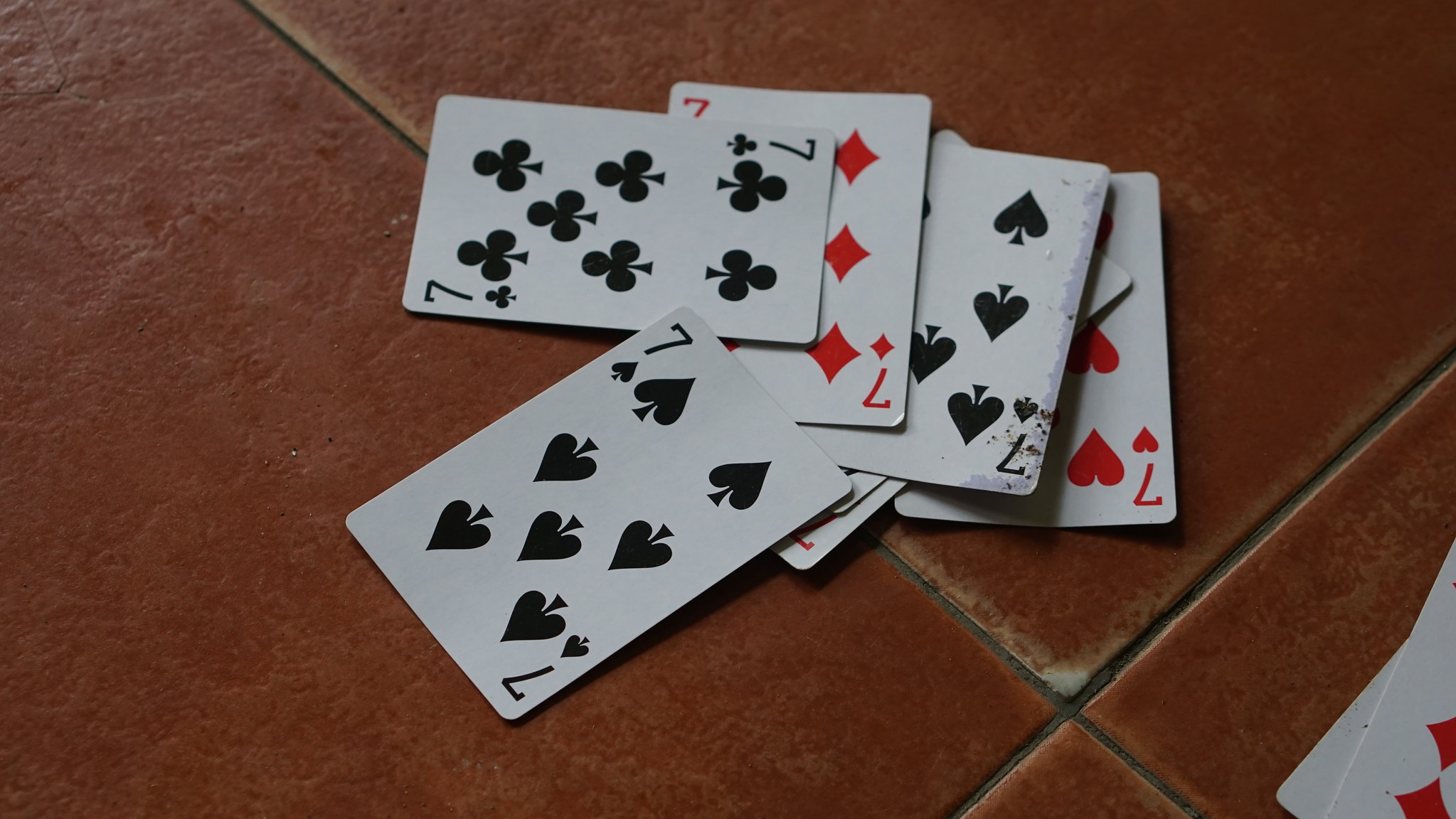The photograph showcases a collection of playing cards neatly arranged on a slightly worn, terracotta-colored tiled floor. The tiles' grout is a dark gray, and signs of wear are visible along the edges. Dominating the center of the image is a carefully stacked pile of cards, each one featuring the number 7. This deck includes all four suits: hearts, diamonds, spades, and clubs, presenting a mix of red and black colors. Notably, there are seven cards in this central stack, emphasizing the numerical theme. In the bottom right corner of the photo, two more cards are visible, with the top card being a red diamond. Only a small portion of the white card beneath is exposed, hinting at the layered composition.